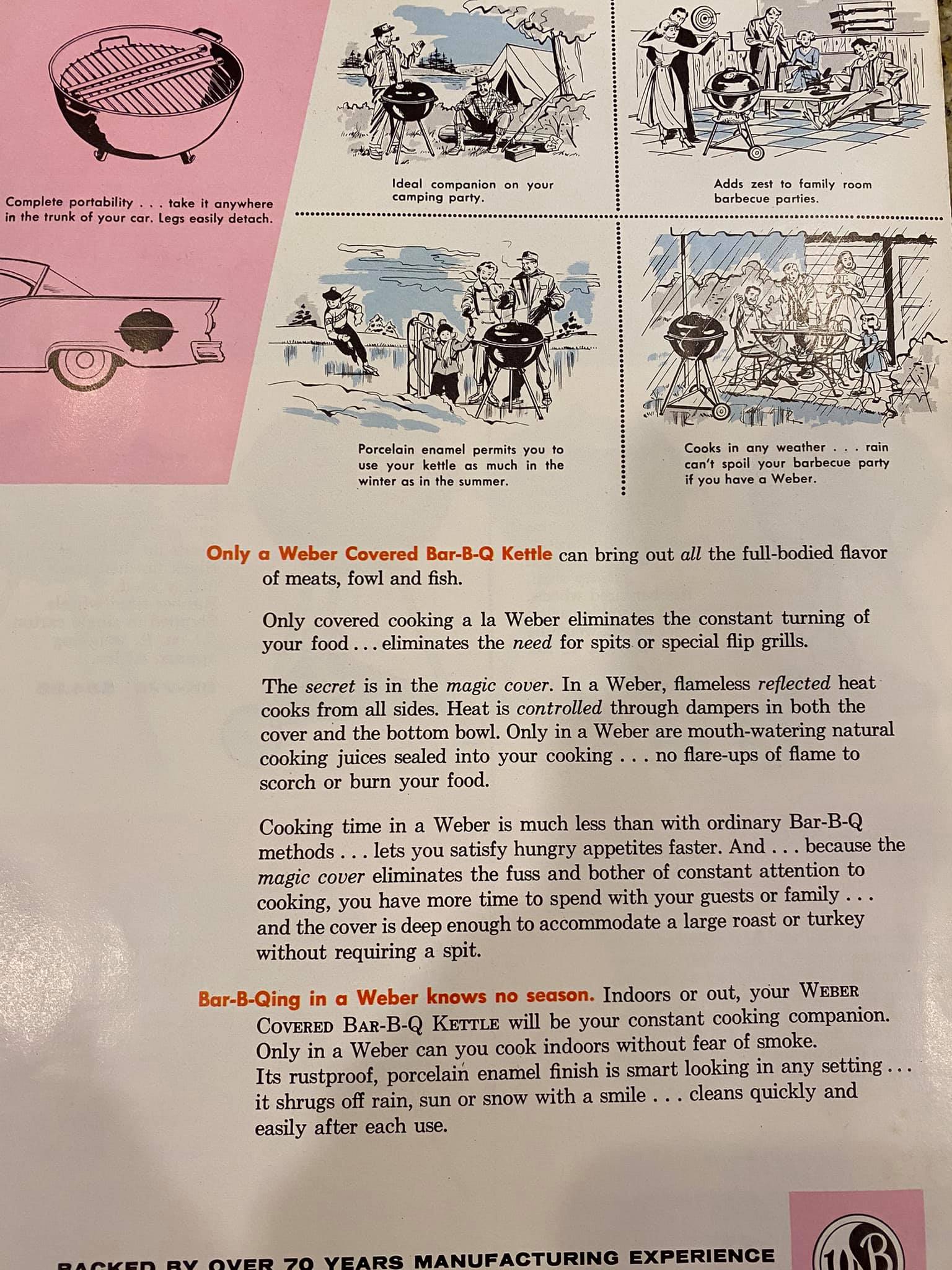This advertisement, seemingly from the 1950s or 60s, extols the virtues of the Weber covered barbecue kettle. The top of the ad features several images showcasing the grill in various settings: a campsite with two men, an outdoor party, a family under an awning during a rainstorm, and a winter scene with a family ice skating. Each scenario emphasizes the grill's versatility. 

A small pink square on the left highlights the kettle's complete portability, noting that the legs easily detach and it can fit into the trunk of a car. Below, detailed text explains that the secret to the Weber's superior cooking is its 'magic cover,' which uses flameless reflected heat to cook from all sides, sealing in natural cooking juices and preventing flare-ups. The heat is controlled through adjustable dampers on both the cover and the bottom bowl. This method reduces cooking time and eliminates the need for constant attention, allowing more time with family and guests. 

The kettle can accommodate large roasts or turkeys without a spit, is suitable for indoor use due to its smoke-free operation, and features a rust-proof porcelain enamel finish, making it durable in any weather. The ad concludes with the assertion that the Weber grill, backed by over 70 years of manufacturing experience, will be a constant cooking companion in any season. The company logo, in pink, black, and white, appears at the bottom.